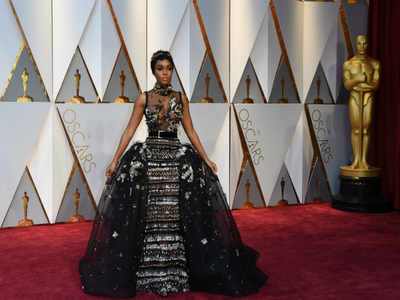The photograph captures a striking moment on the red carpet at the Oscars, featuring a beautiful African American woman, likely a celebrity or actress. She is adorned in an elaborate black dress that dramatically flares out at the hips, in a style reminiscent of Cinderella. The skirt has a unique, intricate design with contrasting horizontal stripes of various shiny materials, making it both eye-catching and elegant. The bodice of the dress is semi-transparent with delicate floral appliques, revealing her arms and accentuating her grace. Her hair is either short or elegantly pulled back, complemented by a matching neck covering or scarf. The backdrop is decorated with "Oscars" text and triangular patterns, and prominently features a large golden Oscar statue on a black stand. Photographers off-frame are undoubtedly capturing her poised and ethereal presence as she stands amidst the glamorous setting.